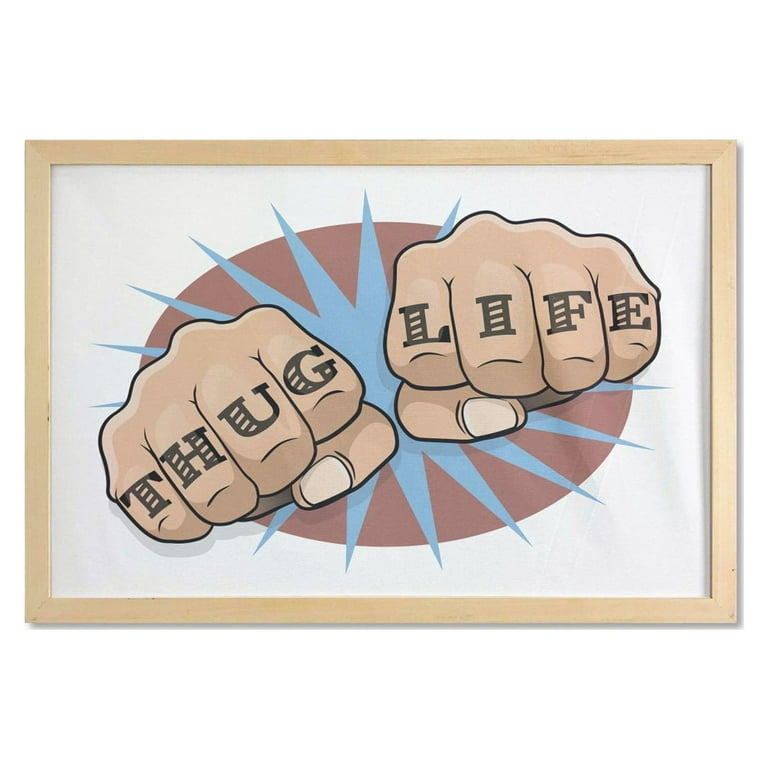A framed piece of art with a light brown, bamboo-like frame occupies the entire image. The artwork features a white background, with a central brown oval overlaid by a blue starburst pattern, reminiscent of a spiked word bubble from a comic book. Emerging from the center of this design are two cartoonishly drawn fists with thumbs tucked underneath, depicted in a flesh color. On the knuckles of the right hand, the letters "T-H-U-G" are inscribed in black with white insets, and on the left hand, the letters "L-I-F-E" appear in similar style. The fists and the lettering create an impression that the words "THUG LIFE" are tattooed across the knuckles. This horizontal image emphasizes the dynamic contrast between the dark pink, brown, and blue-toned background elements and the impactful message on the fists.